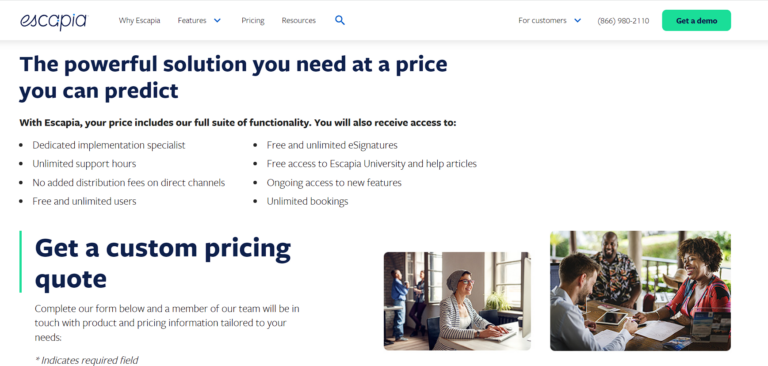This is a highly-detailed screenshot of the "Escapia" website homepage. At the top of the page, there is a banner with the text "Why Escapia?" and a navigation menu offering options such as Features, Pricing, Resources, a search icon, a link for Customers, a phone number, and a prominent green button labeled "Get a Demo."

The main section of the page features the headline "Powerful solution you need at a price you can predict," emphasizing Escapia's comprehensive offerings. Below this headline, the site specifies that the price includes their full suite of functionalities. Additionally, there are eight bullet points detailing the specific benefits and features included in their offer.

Further down, another headline in large blue text reads "Get a custom pricing quote." Below it, there's an invitation to "Compare our form below, and a member of our team will be in touch with product and pricing information tailored to your needs." Next to this is an icon or asterisk indicating that certain fields are required.

To the right of this text, there are two images. The first image shows a woman sitting at a computer while two people converse behind her. The adjacent picture depicts three people sitting at a desk, engaging in animated conversation and laughter.

Overall, the webpage combines informative text with relatable imagery to convey the user-friendly and comprehensive nature of Escapia's services.